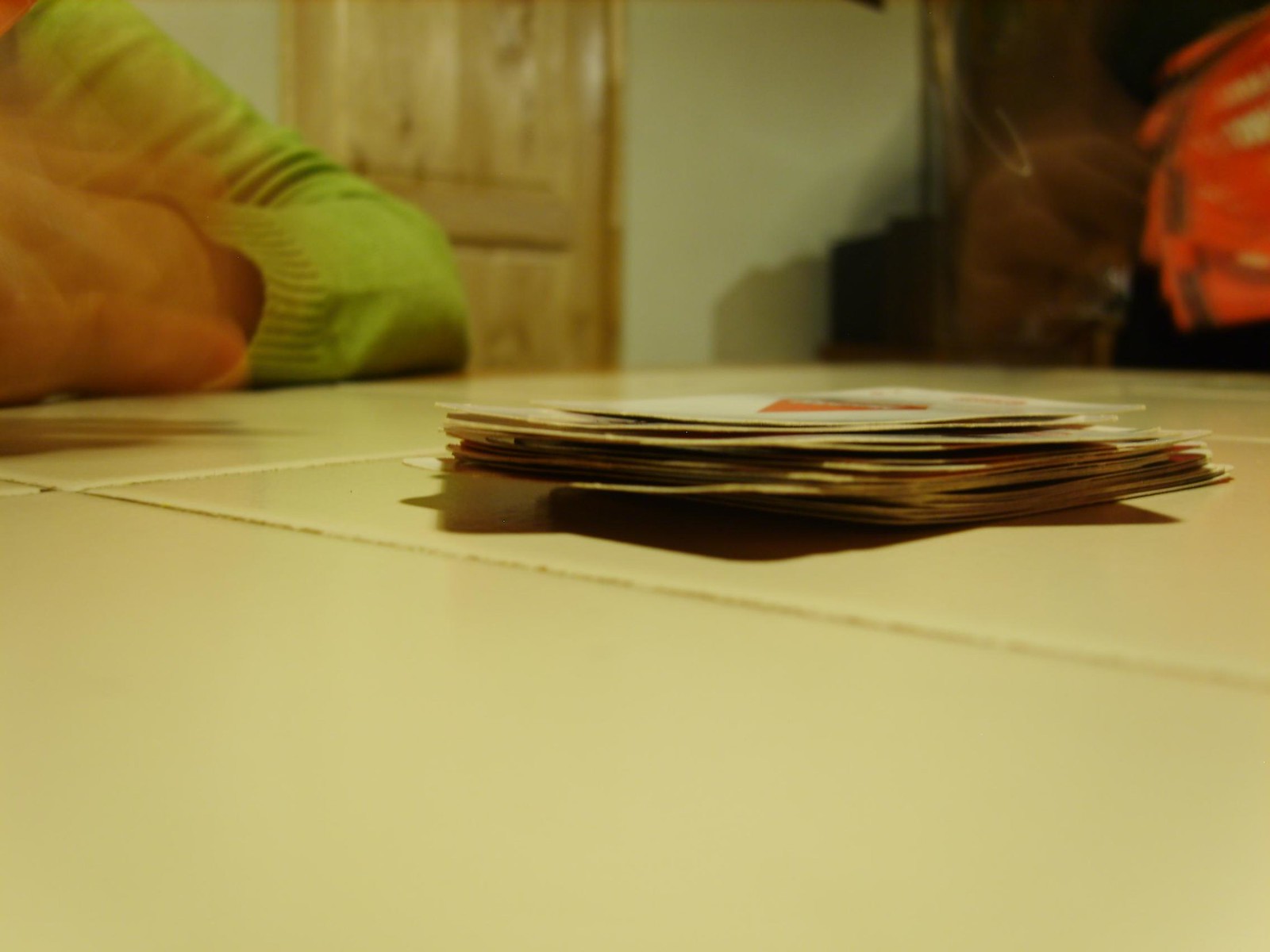In this photograph, there is a weathered stack of cards, possibly playing cards or game cards, resting on a tiled surface. The stack appears thin and buckled, with the cards showing signs of age as their edges are dirty and frayed. The top card features a faint red object that is difficult to discern. The tiles beneath the cards are yellow or ivory and appear to need some re-grouting. 

A person in a long-sleeved, apple-green sweater is seated at the tiled surface, with their forearms resting on it. Their left hand is reaching toward the cards, captured in a motion blur. In the background, an off-white wall extends to a wooden door. To the right of the wall, there is a blurry image that appears to be a stack of jackets or possibly a backpack on a chair. The overall scene suggests a sense of casual disarray and age.